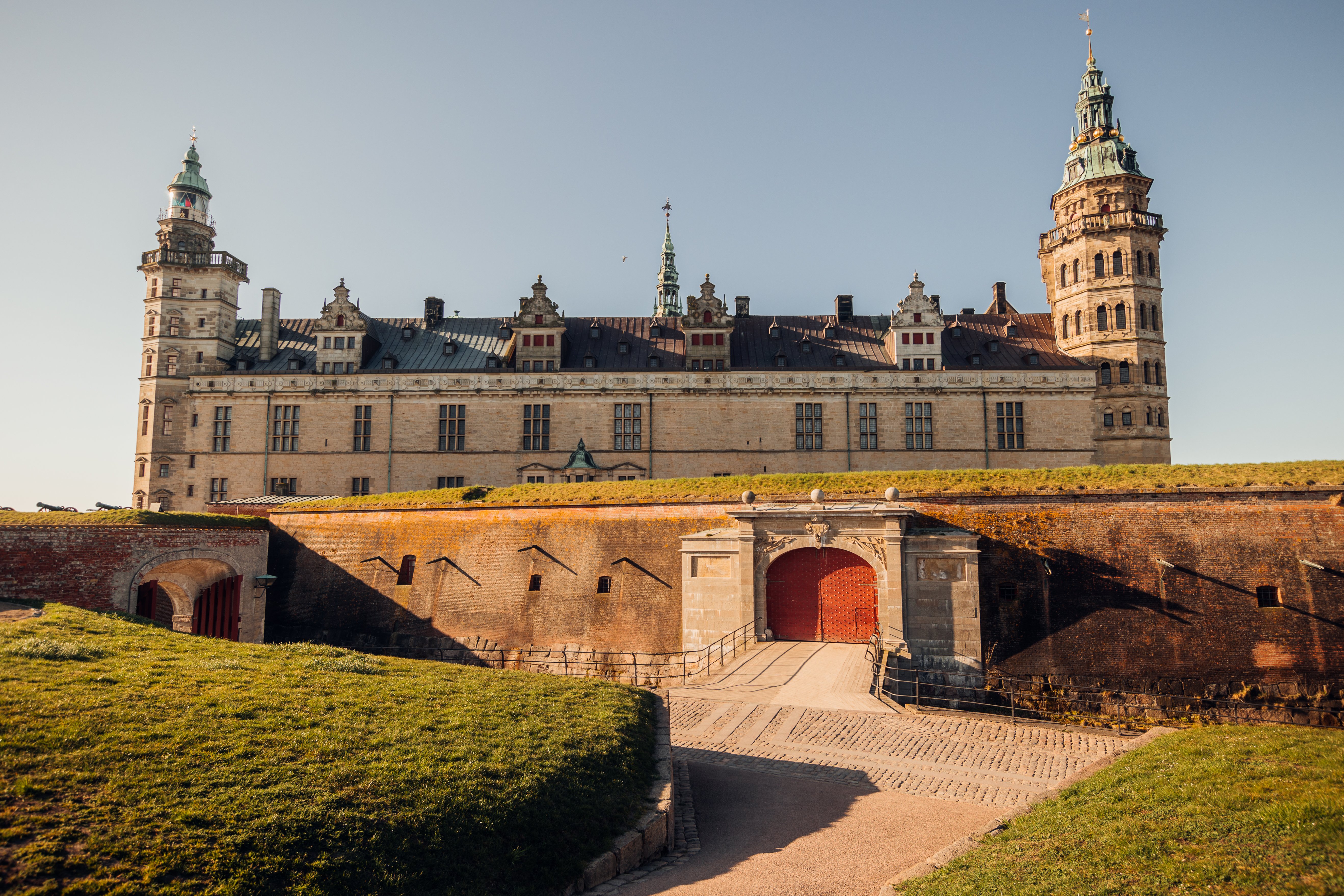The photograph captures an expansive view of a historic European castle, likely the famous Hamlet castle in Denmark. Taken in full color on a clear, cloudless day, the photo features natural light with muted, non-vibrant tones. The foreground is adorned with well-maintained grass and thick shrubbery, which occupy both the bottom left and right corners of the image. A beige sidewalk, likely made of stone, cuts through the center, flanked by greenery and leading towards the castle.

The castle itself dominates the center of the composition and spans most of the image's width. Its exterior is a beige hue, punctuated by numerous windows. Two prominent towers stand at each end; the left one features a pointed roof cap, while the right tower, which boasts five layers, is crowned with a statue. Elaborate dormer windows with pointed ornaments punctuate the dark brown shingled roof. An ornate, arched stone gateway with red double doors provides entry to the castle grounds, with an iron fence positioned before the heavy, likely locked, orange castle door in the distance.

Above the castle, the sky is a pristine blue, framing the scene in serene, natural light. This composition, viewed from ground level looking slightly upwards, imbues the scene with a grandeur reminiscent of a richly detailed stately home, calling to mind the iconic Downton Abbey. A subtle radio tower peeks from the center, adding a touch of modernity to the timeless structure. The photograph offers a detailed and lifelike representation of this majestic and storied castle.